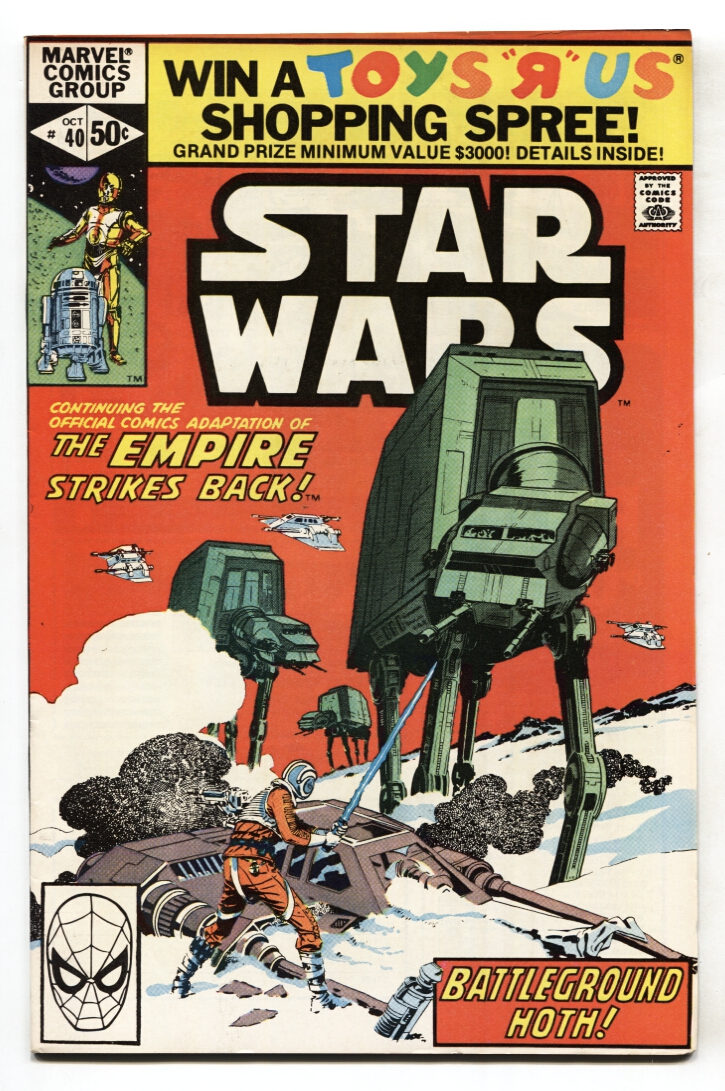This image depicts a vintage cover of a Star Wars comic book from "The Empire Strikes Back" era. The piece is vertically rectangular with no specific border or background. Prominently placed at the top, a yellow banner announces, "Win A Toys R Us Shopping Spree, Grand Prize Minimum Value $3,000." On the upper left corner, the Marvel Comics Group logo is displayed alongside illustrations of C-3PO and R2-D2. The title "Star Wars: The Empire Strikes Back" stretches across the top, set against a backdrop featuring the icy planet of Hoth. A dramatic scene unfolds below: Luke Skywalker, wielding his blue lightsaber, confronts the towering AT-AT walkers. In the lower left corner, there is a black and white image of Spider-Man, and the lower right corner contains the words "Battleground Hoth." The artwork and coloring evoke a nostalgic feel, reminiscent of vintage comic book styles.